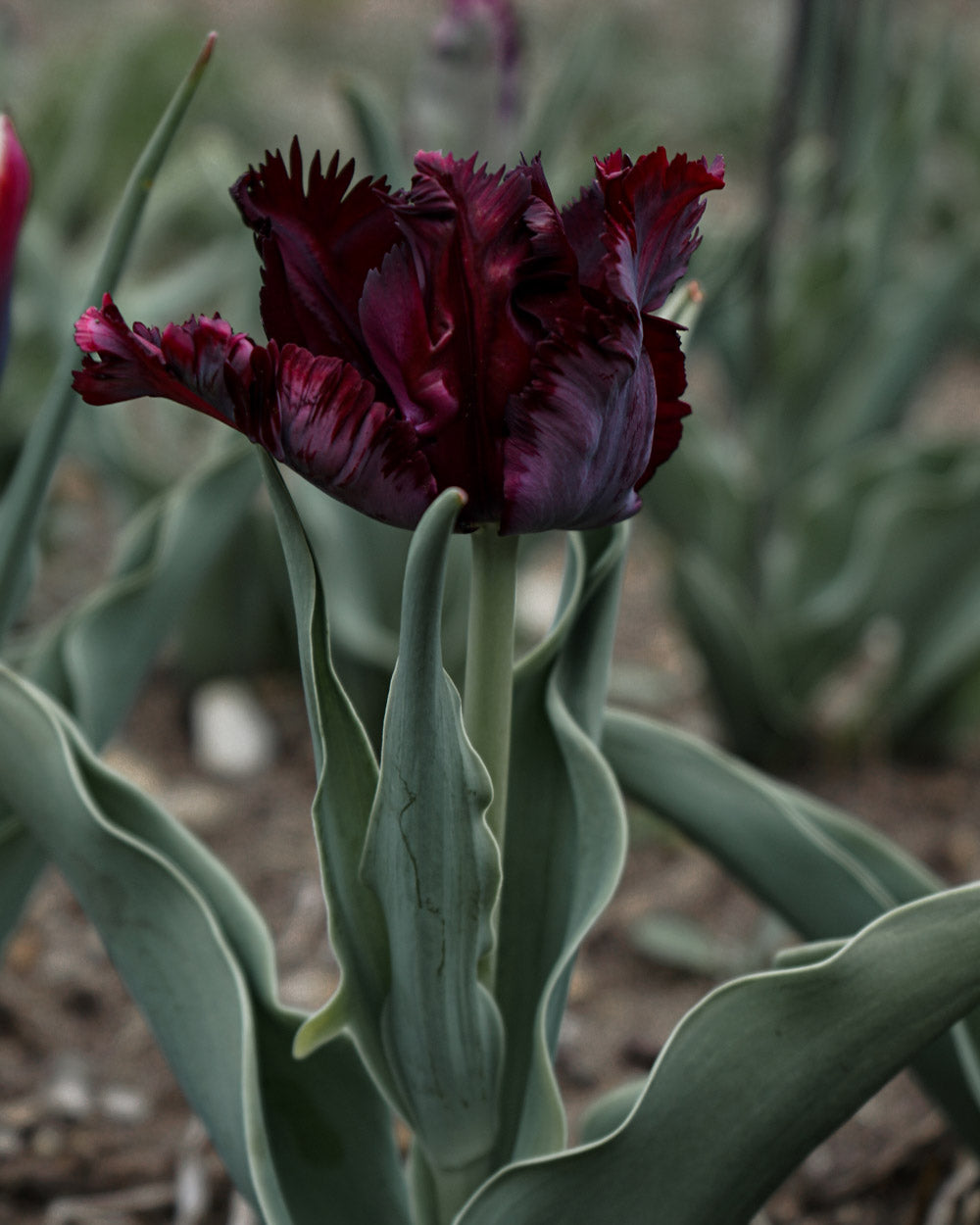In this striking image, the main focus is on a single, dark red flower with a stunningly rich blood-red hue, bordering on burgundy. The flower’s delicate petals are ruffled and serrated, giving them a rounded yet spike-like appearance that contrasts beautifully with their velvety softness. The flower, which appears almost black under the subdued lighting, occupies the top third of the image. The stem and leaves below are a sage green, lighter in tone, and display a velvety texture that matches the flower. The edges of the leaves showcase a wavy pattern and surround the green stem. The background, blurred and muted with a possible filter, hints at an entire field of similar flowers, their emerald green leaves slightly tinted with white, contributing to the overall soft and ethereal ambiance of the scene. אינt the top left corner, a subtle glimpse of another flower adds depth to this quietly dramatic composition.